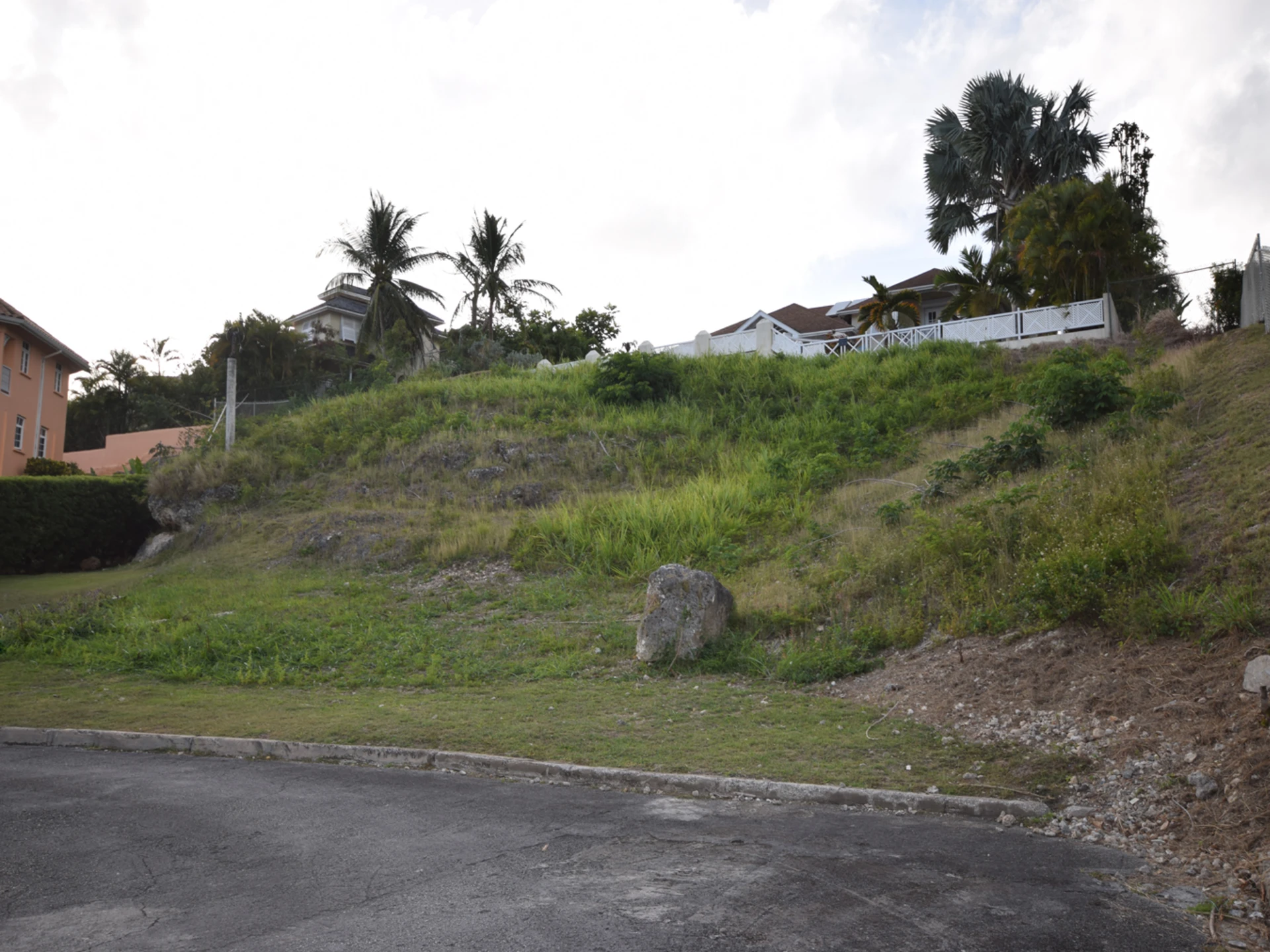In the foreground of this outdoor scene, a paved street with a gray curb runs horizontally. Beyond the street, a grassy hill begins with short, patchy grass and gradually transitions to taller grass as it ascends. A large gray boulder is prominently situated near the bottom center of the hill. The hill also features some dirt patches and green bushes.

On the left side, a two-story, light orange or salmon-colored house stands next to neatly trimmed bushes. As the hill slopes upward, various upscale houses are partly obscured by the terrain and abundant tall palm trees. A white fence runs across the hill's right side, partially enclosing another house with a brownish roof that peeks out from behind more palm trees.

The sky above is filled with thick white clouds, with small patches of blue visible in between. The overall setting hints at a tropical or upscale residential area, rich in greenery and architectural detail.